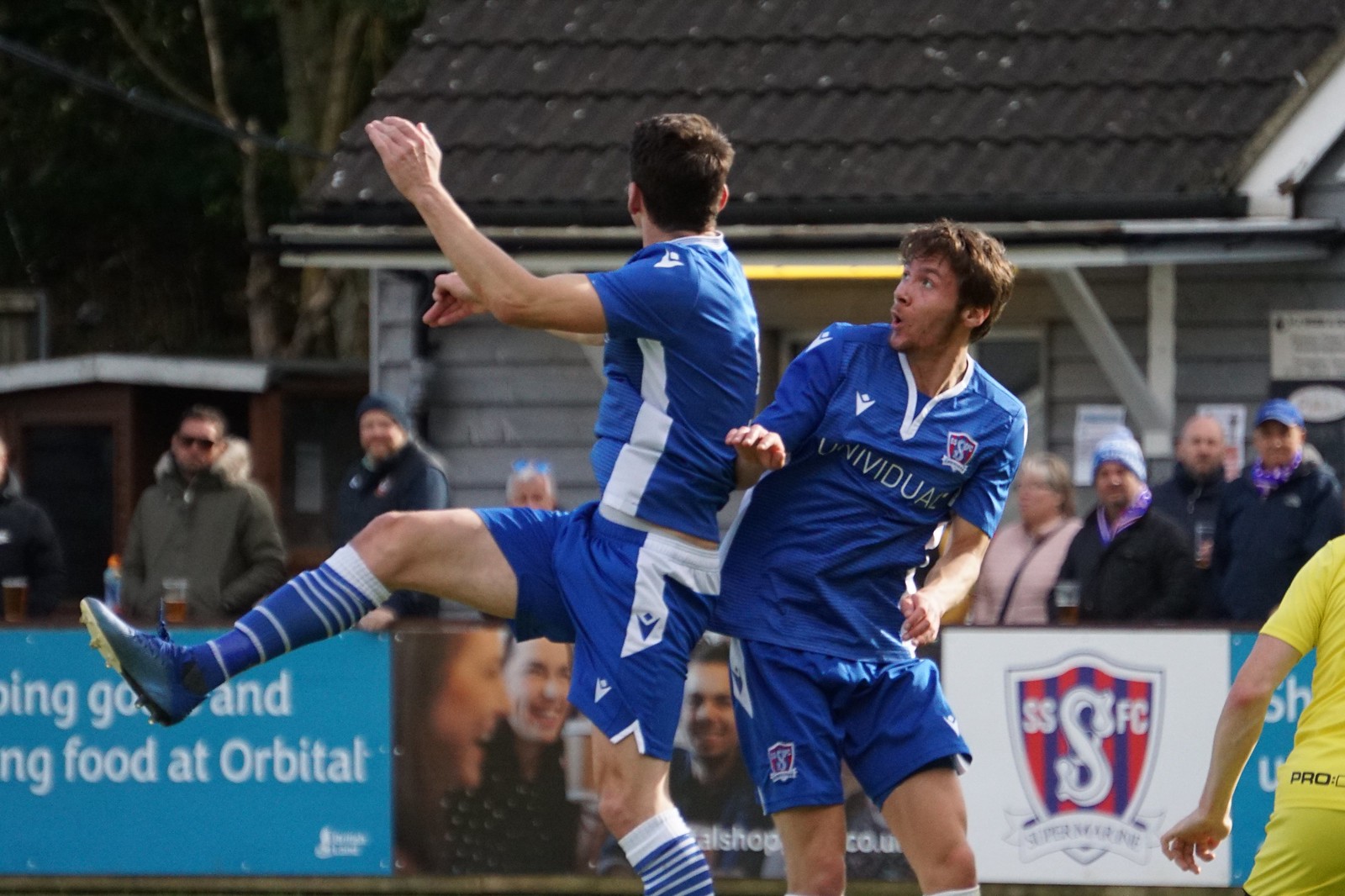In this detailed action shot from a rectangular soccer game photograph, two players in blue uniforms with white trim are captured mid-play against a backdrop of spectators and advertisements. The player on the left, whose right leg is airborne with his left foot planted, is looking towards the right, showcasing his blue socks with white stripes. The other player, positioned slightly behind, is facing the camera and looking up to the left, likely tracking the ball. Both are wearing blue jerseys and shorts. In the bottom right corner, a partially visible player in a yellow uniform can be seen. Behind the players is a boundary lined with various sponsor banners, including partly legible texts like "food at orbital" and "SSFC." Spectators, bundled up in heavy coats and winter hats, stand beyond the boundary. Further in the background is a small building, potentially a concession stand, featuring wood planking, horizontal green stripes, a dark tiled roof with an overhang, adding depth to the scene.